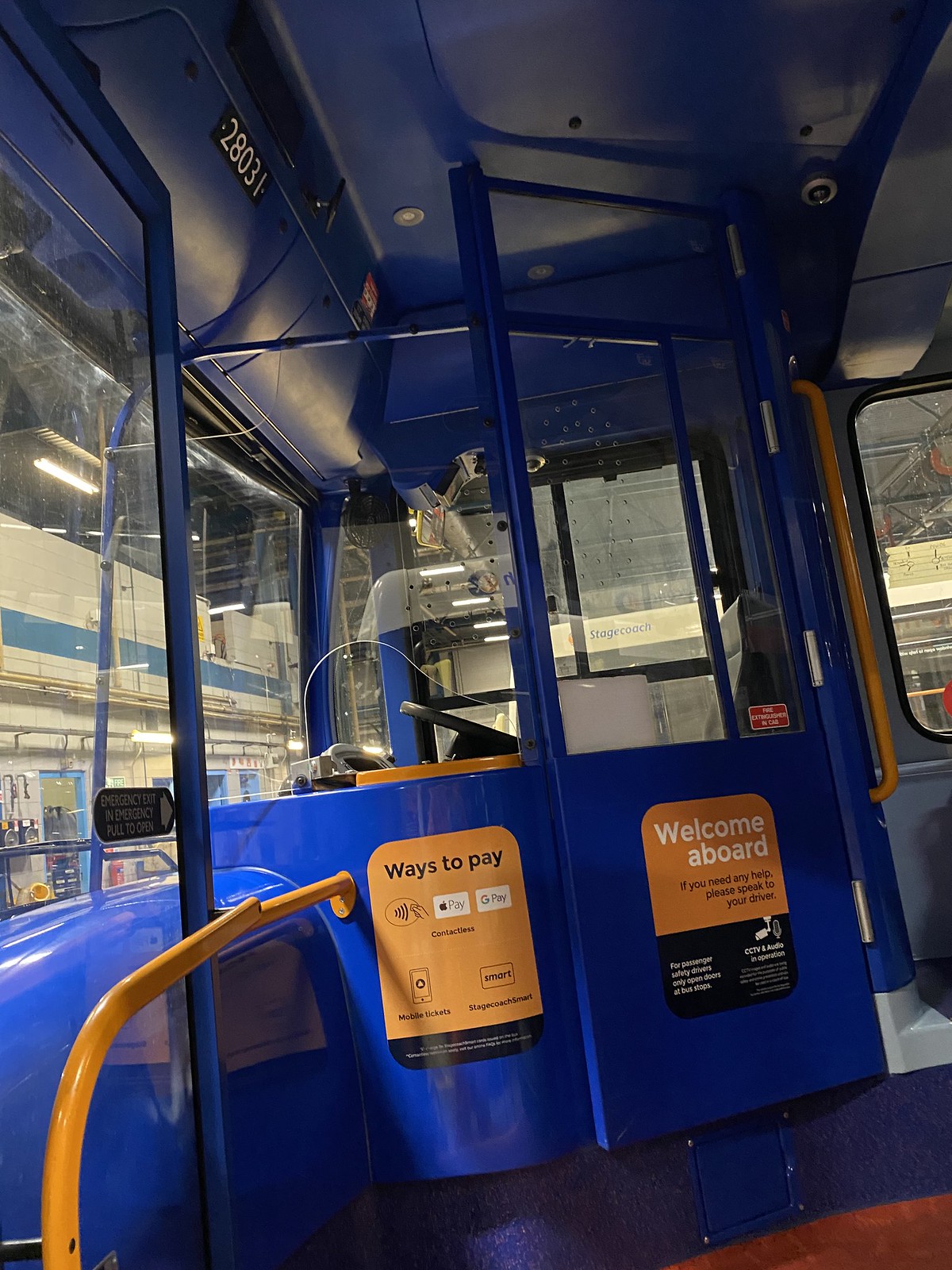The photograph, taken inside of a bus parked within a garage, showcases a predominantly blue interior, including the ceiling, walls, and driver's area. The driver's cabin is enclosed with blue panels and features a plexiglass top with a small arched opening for fare transactions. A black steering wheel and chair are visible within the cabin. On the left side, there is an orange handrail and two orange signs. One sign, with text detailing the payment methods available including Apple Pay and Google Pay, reads "Ways to Pay". The second sign, split into orange and black sections, says "Welcome Aboard" and instructs passengers to speak to the driver if they need assistance. Near the ceiling, the bus number 28031 is displayed prominently.